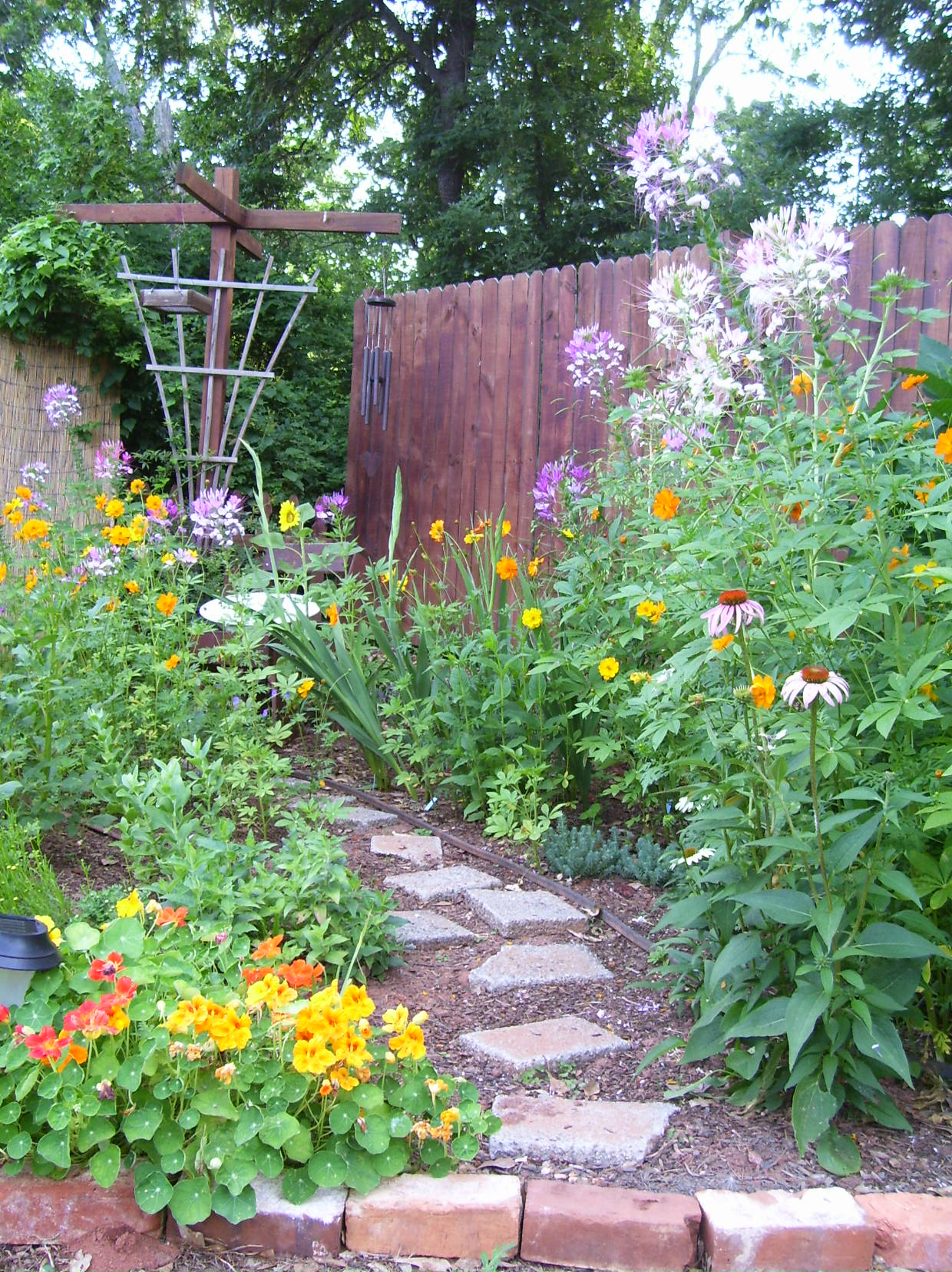This photograph showcases a charming and meticulously managed backyard garden. The centerpiece is an irregularly shaped stone walkway, composed of individual stone blocks spaced by patches of dirt, leading to a bird bath at the far end. Both sides of this quaint path are adorned with a diverse array of vibrant flowers in a natural arrangement, featuring shades of yellow, pink, purple, orange, and white. Among the flora, tall flowers and greenery create a lush backdrop, including mixed white and purple blooms, black-eyed Susans, and nasturtiums.

To the side, a wooden trellis completes the picturesque scene, adorned with a wind chime and acting as a potential support for climbing plants or a perch for bird feeders. A lattice likely serves the same purpose, enhancing the garden's charm with its potential for floral growth. Adding to the serene atmosphere, a small fountain and garden lights are thoughtfully placed within the space. The flower beds are bordered with bricks, giving a tidy yet vibrant touch to this spring garden oasis.